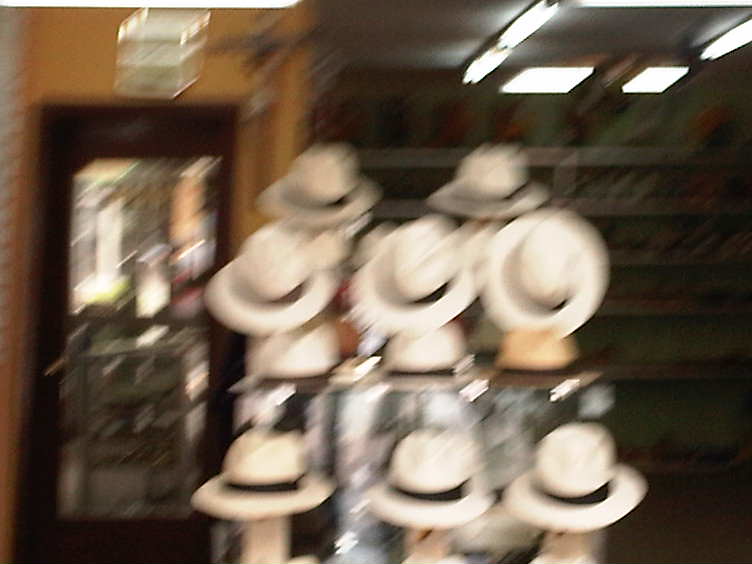This incredibly blurry photograph captures what appears to be the inside of a hat shop or a men's clothing store. Due to the out-of-focus and shaky camera, the image is difficult to discern, but it prominently features a collection of high-quality straw hats, resembling fedoras, with black or dark gray bands encircling the crowns. Arranged on a multi-level display stand, there are three hats on the bottom level facing away, another three laying flat on the shelf above, and two more at the top facing downward. The background is predominantly dark, with shades of black and brown, and includes a brown-framed door, possibly with a mirror or window, and some ceiling lights, likely fluorescent. The entire scene is marked by blur lines at a 45-degree angle from lower left to upper right, making the details almost indistinguishable but hinting at metal shelving and bracketed items in the store.